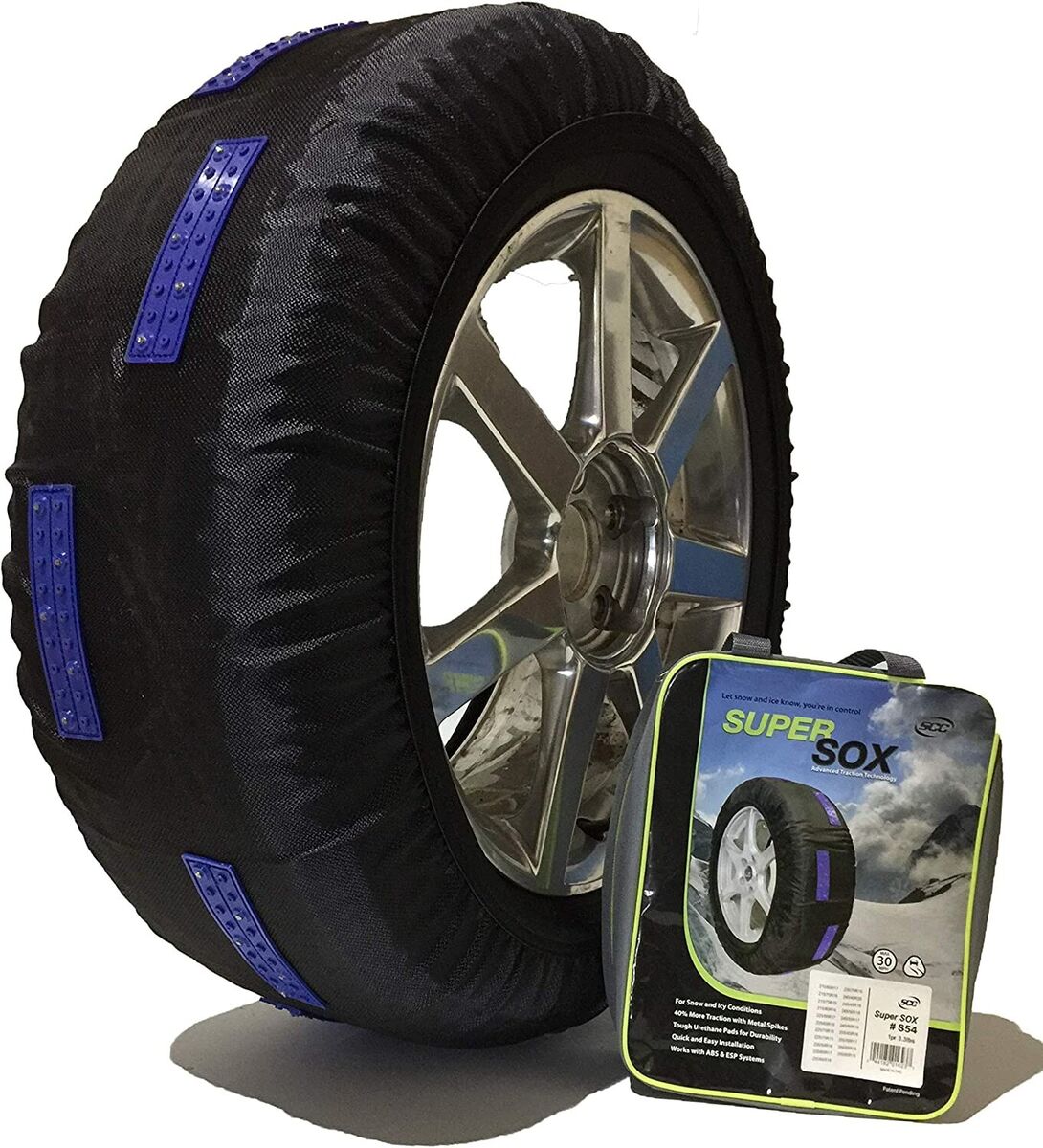This image features an advertisement for a product called "Super Socks," designed to improve tire performance in snowy conditions. At the center is a large, diagonally positioned, brand-new tire with a chrome, star-patterned rim. The tire is wrapped in the Super Socks product, which consists of a black fabric with blue strips of gripping material to enhance traction on snow. The background is stark white, making the colors of the product—black, blue, silver, and white—stand out prominently. Below the tire, towards the bottom right, is the product's packaging. The packaging displays "Super" in mint green text and "Sox" in black text, alongside a rotated image of the tire. Both the tire and the package cast subtle shadows, adding depth to the clean, minimalist design of the advertisement.